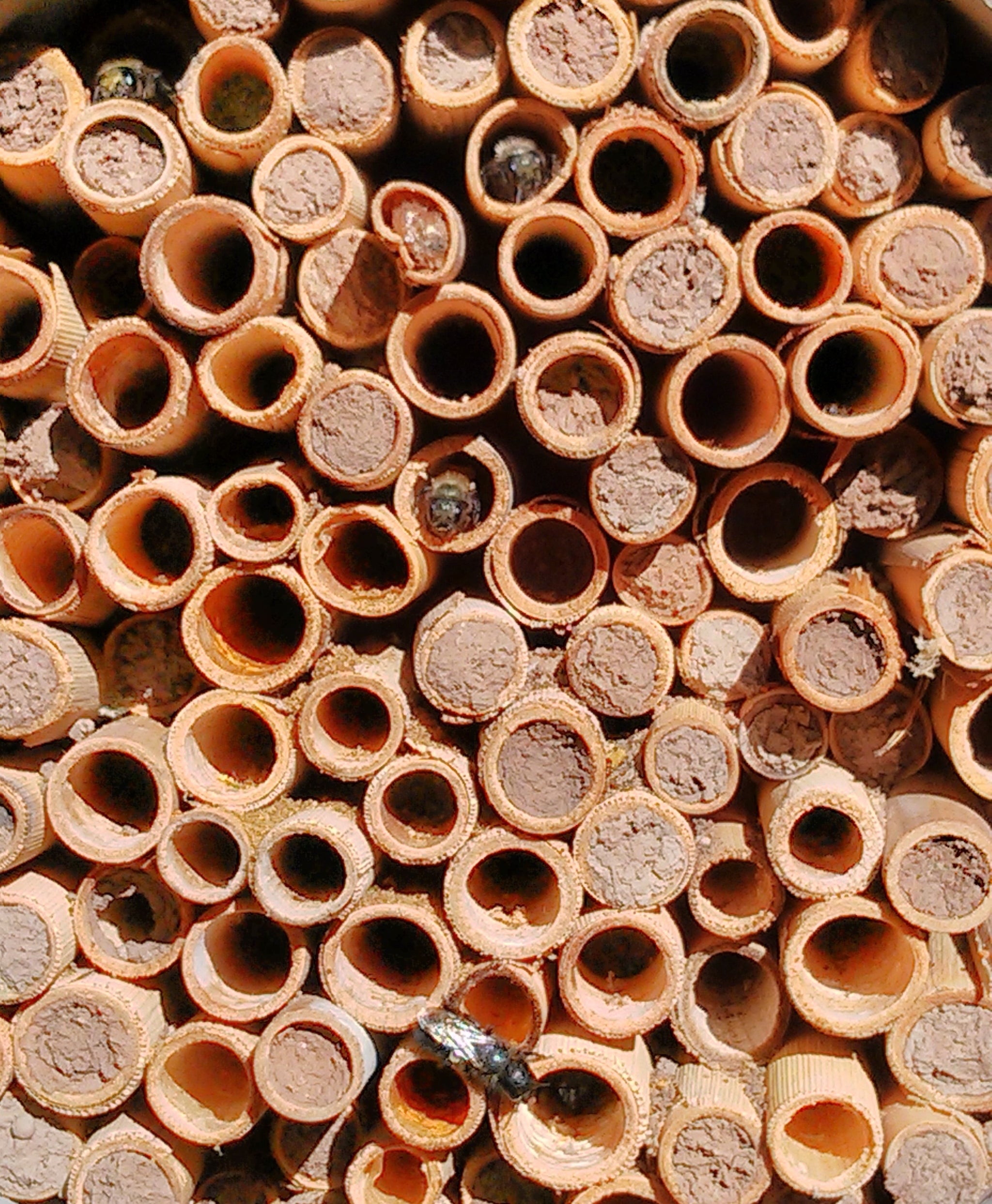The image is a vertical, rectangular snapshot that closely resembles an array of terracotta cylinders, or hollow tubes, standing both horizontally and vertically. These tubes have a brownish exterior, transitioning to an orange hue on the inside and ultimately turning black at their deepest point. Scattered among the tubes, some are filled with a substance akin to mud or clay, while others remain empty. There are multiple bees present – some perched at the entrances, their heads emerging from a few of the tubes, and others visible within the open spaces. Although it resembles the structure of a beehive, the material inside does not appear to be honey but rather looks like clay, indicating a possible makeshift habitat or an outdoor project related to bee rehabilitation. The scene is brightly lit by intense sunlight, with the black background highlighting the varying contents and bees within the tubes. There is also another smaller insect visible at the top of the image.